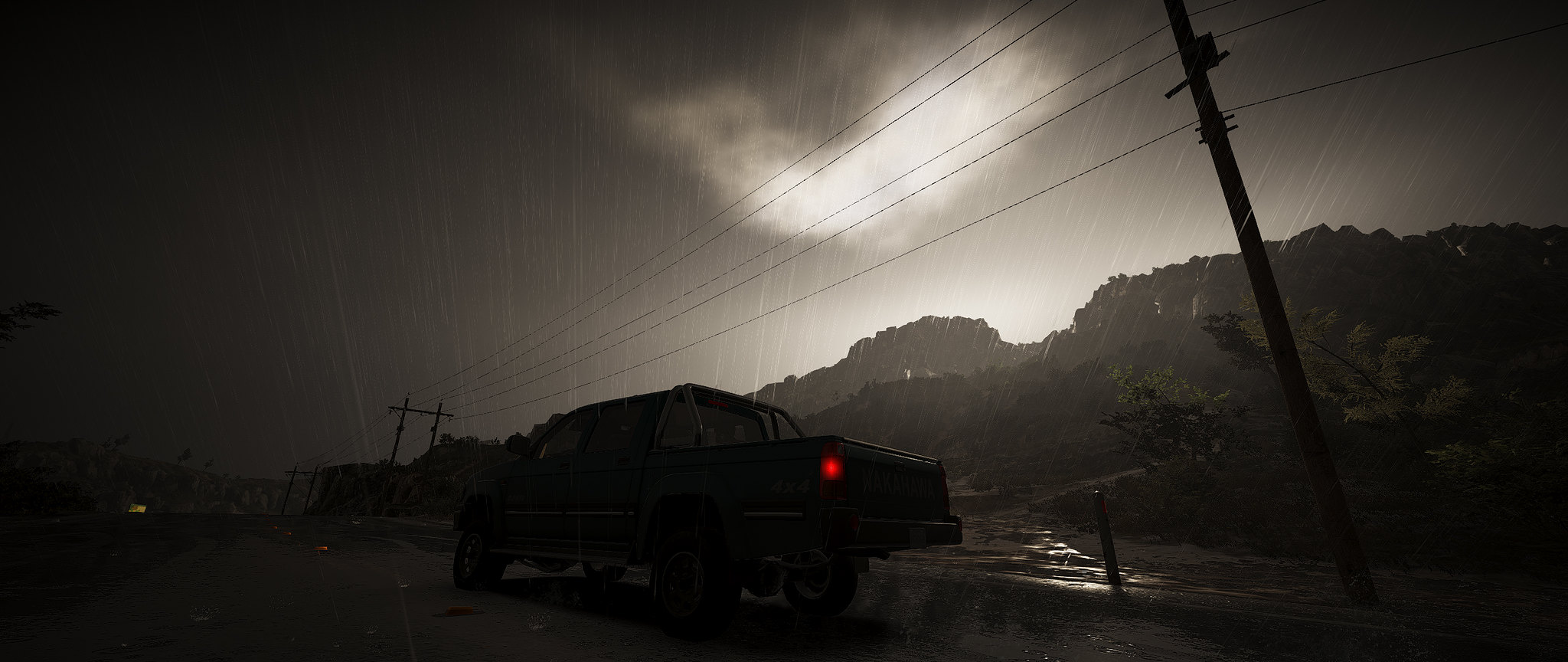This detailed caption describes a surreal and somewhat uncanny scene that may be either a screenshot from a high-resolution video game or an AI-generated image. At the center of the image, in the lower portion, is the silhouette of what appears to be a military-type vehicle, possibly a jeep or a pickup truck with a roll bar. Its square back and the glow of a red taillight add to the realism of the scene. Above the vehicle, the sky looms stormy and turbulent, suggesting a nighttime thunderstorm with heavy rainfall. The horizon is lined with trees, illuminated by a mysterious light that casts reflections on the muddy, rain-soaked terrain.

Amidst the rain, which is falling heavily, there is a slanted power pole that stands out as incorrect. The power lines run peculiarly across the pole without the typical outward struts or supports, and there is a misaligned crossbar with what seems to be a small transformer or circuit breaker, positioned diagonally—another oddity. In the distance, a double power pole does not align properly within the context of the image, further indicating the possibility of AI involvement or a graphical inconsistency in a video game.

Overall, this scene blends partial realism with unnatural elements, pointing to its origins as either a highly detailed game screenshot or an AI-generated artwork depicting a military vehicle amid a dark, stormy night.